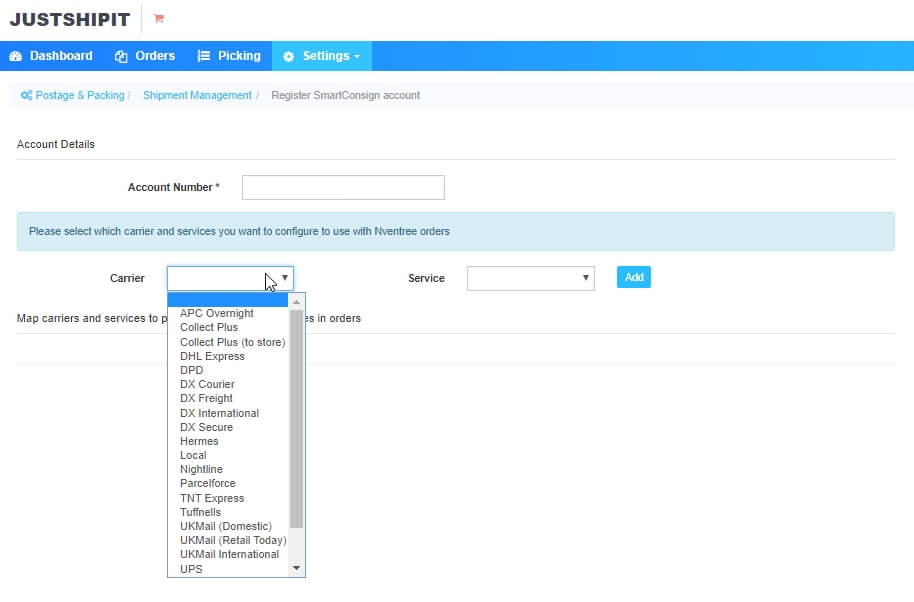This image is a detailed screenshot from the website of JustShipit, an international shipping company. The website features a clean, predominantly white background accented with blue banners and blue text links. The JustShipit logo is prominently displayed at the top, followed by a navigation banner with tabs labeled "Dashboard," "Orders," "Picking," and "Settings," the latter being highlighted to indicate the current page.

On the "Settings" page, the user has navigated through various sections: from "Postage and Packing" to "Shipment Management," finally arriving at the "Register Smart Consign Account" section. This area features a field for entering an account number followed by a prompt that reads, "Please select which carrier and services you want to configure to use with inventory orders."

The screenshot shows a mouse pointer clicking on a drop-down menu labeled "Carrier," which reveals approximately 20 different carrier options for the user to choose from, enabling them to configure their preferred carrier services for shipping inventory orders.